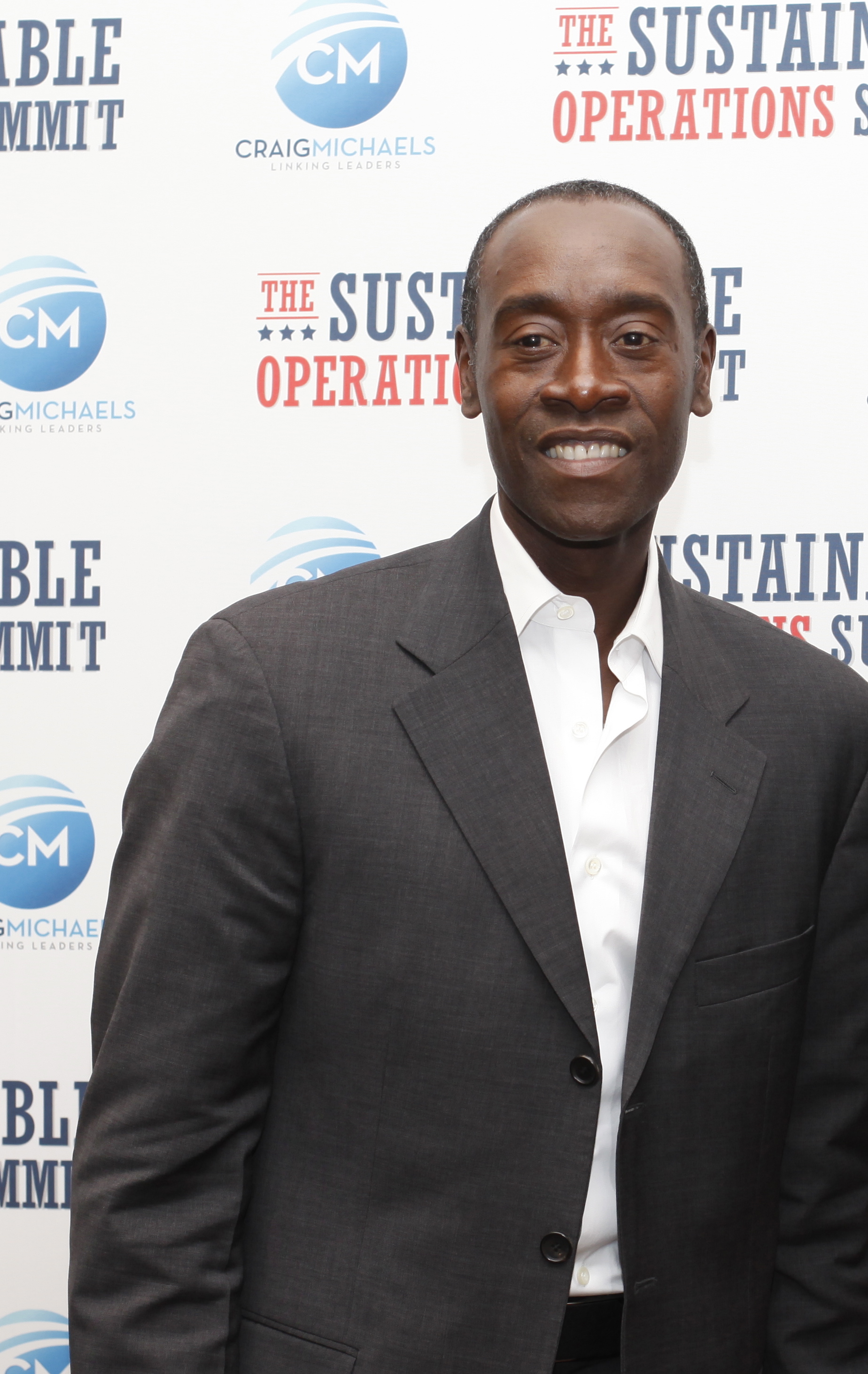In this photograph, an African-American man is smiling and posing in front of a white backdrop adorned with multiple logos and text. The backdrop features a blue circular logo with white stripes and the initials "CM," beneath which is written "Craig Michaels." The background also includes the phrase "The Sustainable Operations" in blue and red, both repeated in a tiled manner. The man, who appears to be middle-aged with thinning black hair, is dressed in a gray suit jacket over an unbuttoned white collared shirt. The suit jacket has two black buttons and a pocket on the left side, with slight wrinkles visible on the sleeves. He is also wearing a black belt. The overall scene depicts the man smiling warmly, highlighting his teeth.